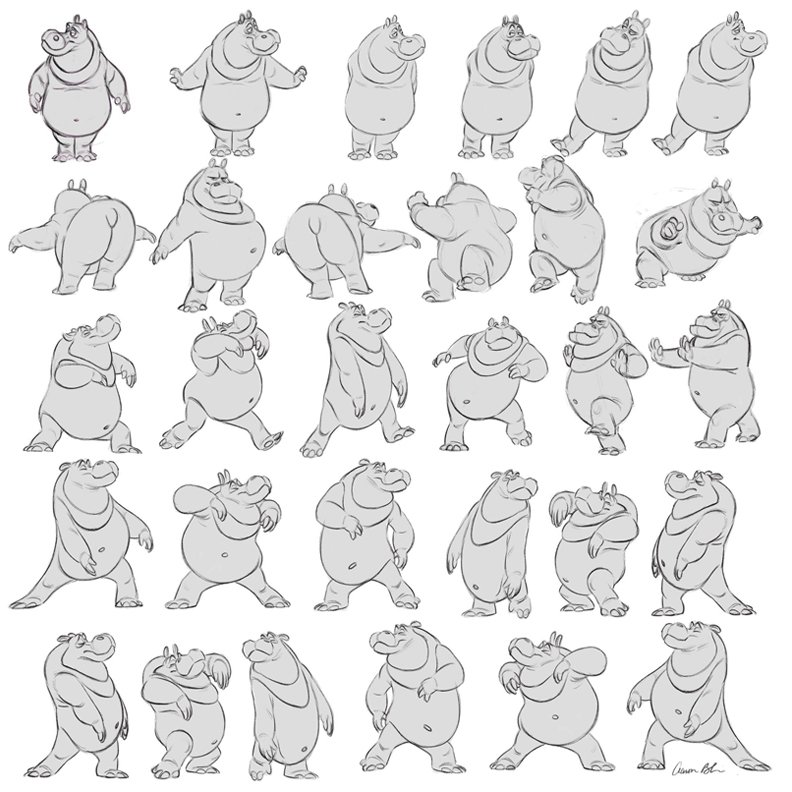This image showcases a portfolio of 30 anthropomorphized hippopotamus character sketches arranged in a grid of five rows by six columns. Each drawing depicts the hippo, notable for its thick neck with an additional fat fold, protruding belly, rounded thighs, short calves, and chunky feet, in various animated poses, creating the effect of different keyframes. The hippo, colored gray with a black outline, is captured in dynamic actions such as standing, smiling, posing, lifting its arms, and dancing, reflecting a sequence of animation stages. The artwork is set against a clean, white background, devoid of any text except for an illegible, cursive illustrator’s signature at the bottom right corner.